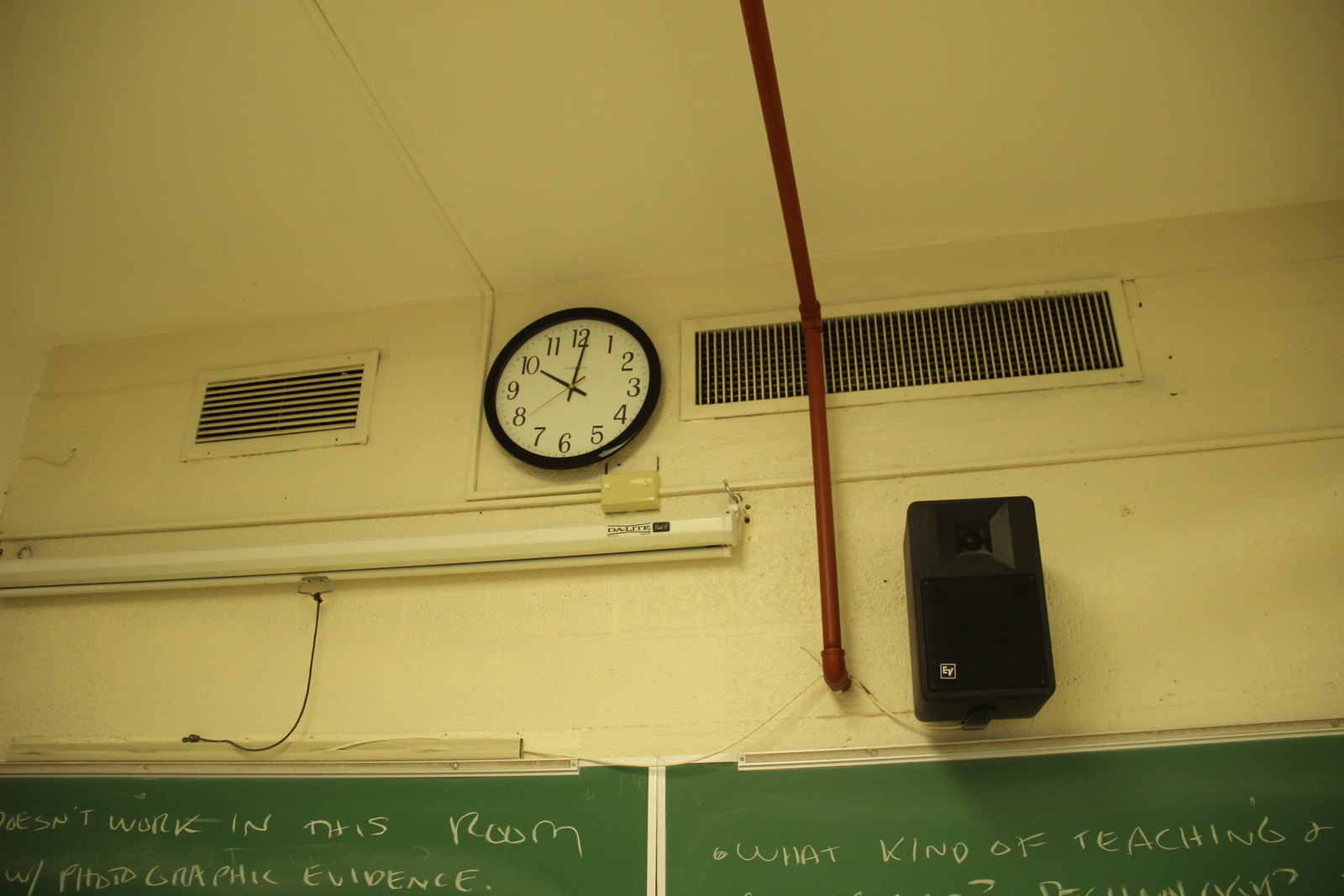The image depicts an older classroom with a distinct, vintage ambiance. The building itself appears aged, evidenced by the weathered, yellowish-white walls. A retracted projector is mounted on the wall, suggesting it is not currently in use. A traditional wall clock with a white face, black numbers, and hands indicating 10:00 with the second hand at the 40-second mark, is prominently displayed. The classroom features two large chalkboards, which are actually green rather than black. Written on the chalkboards are the phrases "Doesn't work in this room" and "What kind of teaching," adding an intriguing element to the scene. Above the second chalkboard, there is a speaker mounted, likely used for classroom announcements. The overall atmosphere brings to mind a bygone era of educational settings.